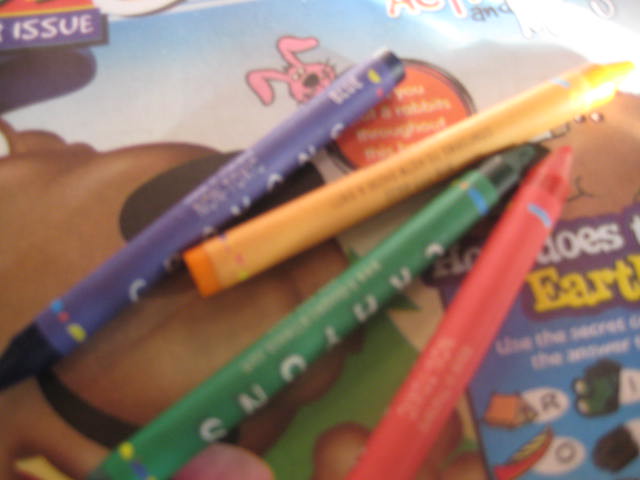This is a close-up, slightly out-of-focus photograph of an activity placemat for children, likely from a restaurant. In the top left, white lettering reads "issue." The placemat features a blue sky background with an assortment of colorful elements: a pink, smiling rabbit in an orange circle, part of a brown dog's face with a black nose and an upturned mouth, a purple crown pointing downwards, a yellow crown pointing upwards, a green crayon, and a red crayon oriented similarly. There are four crayons—blue, yellow, green, and red—arranged diagonally across the placemat. The crayons appear unused or slightly used, with no damage to their wrappers. Scattered on the placemat are various text and images, including partially visible words like "how does" in white, "earth" in yellow, and letters such as "H" and "O." Additionally, there are drawings of a tent and a canoe, enhancing the playful and interactive design of the placemat. Overall, the scene invokes the vibrant, child-friendly atmosphere typical of restaurant activities for kids.